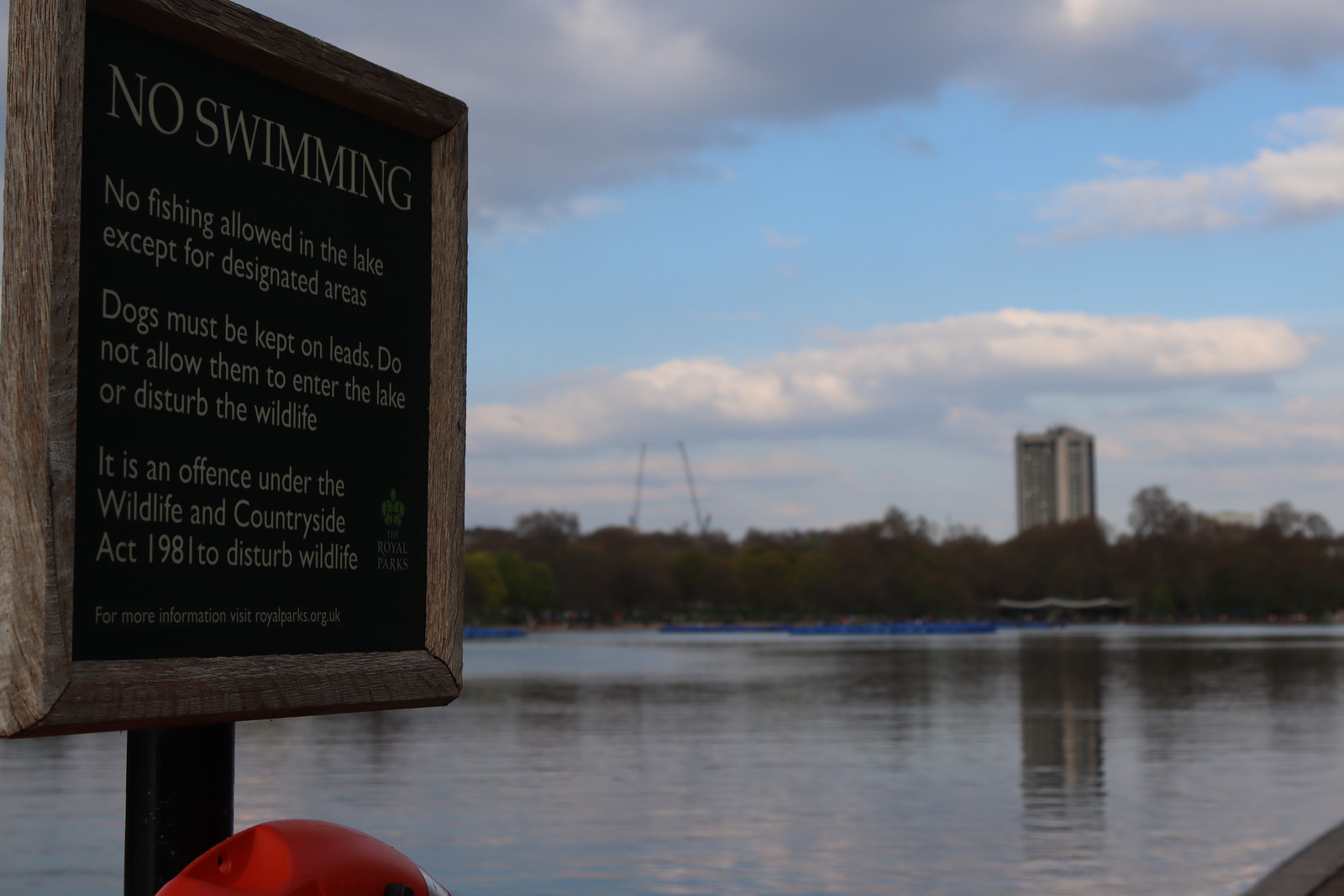The image captures an outdoor scene on a partly cloudy day with patches of blue sky and some grayish-white clouds. On the left side of the photo, there is a black sign with a wooden frame mounted on a metal post. The sign prominently displays in large yellow letters "NO SWIMMING" at the top, followed by "NO FISHING ALLOWED IN THE LAKE EXCEPT FOR DESIGNATED AREAS," "DOGS MUST BE KEPT ON LEASHES. DO NOT ALLOW THEM TO ENTER THE LAKE OR DISTURB THE WILDLIFE," and "IT IS AN OFFENSE UNDER THE WILDLIFE AND COUNTRYSIDE ACT 1981 TO DISTURB WILDLIFE." Towards the bottom, partially obscured by angle, a message about further information directs readers to a website.

In the lower portion of the image, there's a red curved object whose purpose isn't clear. To the right, there's a pool of water that might be a lake or river. Beyond the water, a distant cluster of fairly large trees can be seen, and even further back, a high-rise building emerges on the horizon. Additionally, what appears to be bridge arms that may lift for large ships or barges are visible in the far distance, hinting at a more industrial or navigable waterway. The entire setting suggests a mix of natural and urban elements in the UK.